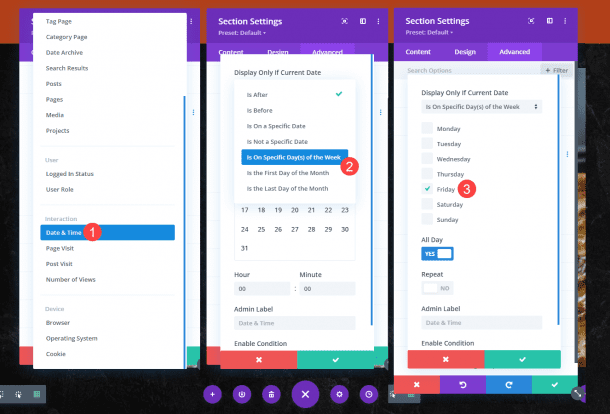This screenshot captures a detailed view of a dashboard interface featuring three side-by-side sections. Each section has a purple header labeled "Section Settings" and includes three white buttons aligned to the right. Below the header, a dropdown menu labeled "Preset Default" is visible. The dashboard is divided into three tabs: "Content," "Design," and "Advanced," each containing step-by-step instructions or settings. On the leftmost section, a menu lists various options with "Date and Time" selected. The middle section displays a calendar interface.